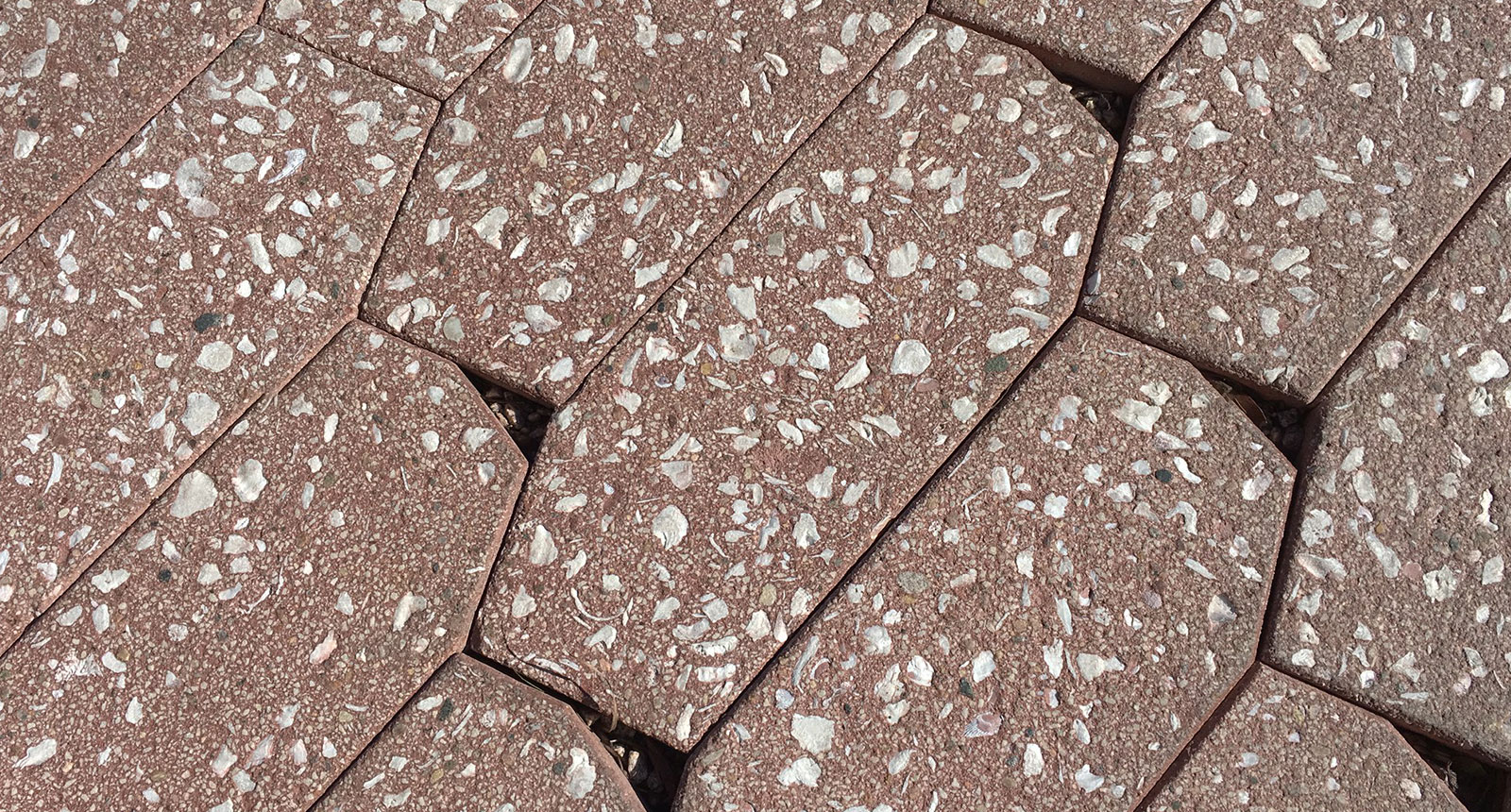The image captures a close-up view of a walkway featuring irregularly shaped cobblestones arranged in a diagonal pattern. Most of these stones, which resemble abstract rectangles with a range of four to more sides, exhibit a brown to tan coloration interspersed with distinctive white speckles and larger white rock fragments embedded within. The cobblestones, about twice as wide as they are tall, create visible spaces between them, revealing small black triangular gaps filled with dirt in certain places. The tightly packed layout shows around twelve individual stones without any text or additional elements, focusing entirely on the detailed texture and arrangement of the cobblestones forming a pedestrian walkway.